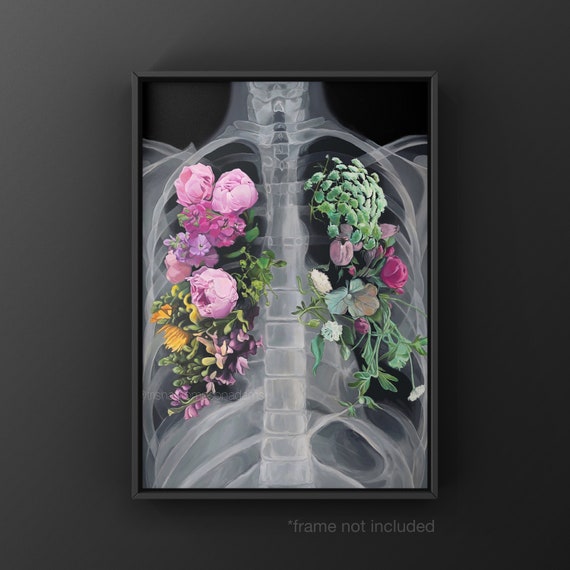The image depicts a rectangular piece of wall art with a simple, modern grey frame, centrally placed against a dark grey background. The artwork resembles an x-ray of a chest, showcasing the spine and light grey rib cage. Where the lungs would be, the rib cage is artistically replaced with vibrant floral arrangements. On the left side, the flowers are primarily pink, encompassing shades from light to hot pink, and are complemented by yellow flowers and green leaves. The right side features clusters of green leaves, interspersed with a central red flower and a few white blooms. The detailed botanical elements are meticulously arranged to mimic the natural structure of lungs, blending anatomical imagery with floral artistry. Text at the bottom of the image notes that the frame is not included.